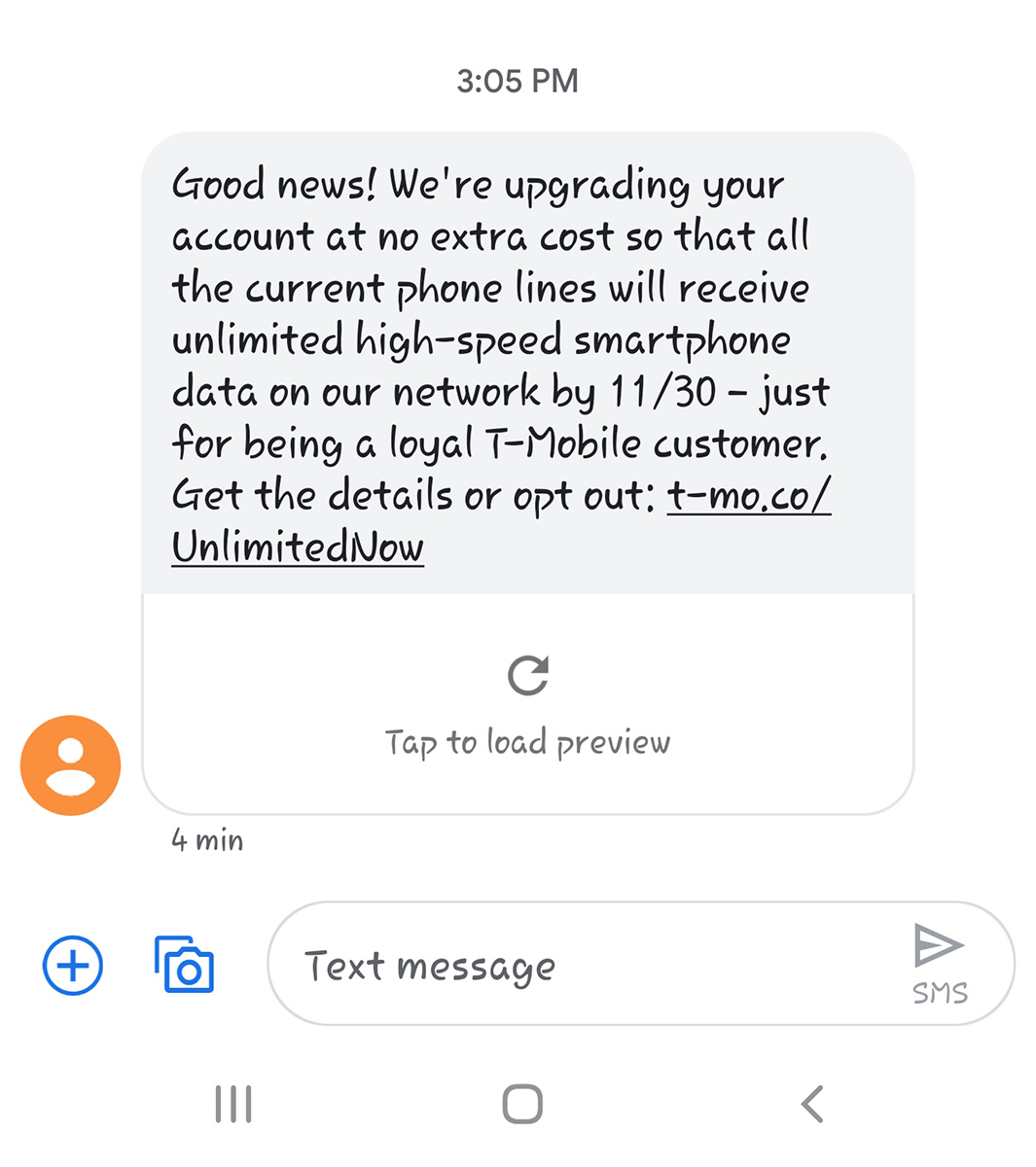This is a screenshot of a text message likely on an Android or Samsung device. The message is displayed in black italic font and reads: 

"Good news! We're upgrading your account at no extra cost so that all the current phone lines will receive unlimited high-speed smartphone data on our network by 11/30- just for being a loyal T-Mobile customer. Get the details or opt-out: t-mo.co/unlimitednow"

The text is set against a light gray background. Below this message, there is a white section with an option that reads "Tap to load preview" in gray text, accompanied by a refresh icon. 

On the left side of the text message, there is an orange circle containing a white person icon. Directly below this, there are two blue buttons: one with a plus sign and the other with a camera icon. 

At the bottom of the screen, within the text message entry field, the placeholder text "Text message" is displayed. On the right side of this field, there is a triangle icon labeled "SMS." 

The navigation bar at the bottom of the screen presents three icons: a vertical hamburger menu (likely representing a menu button), a black or gray square (indicating the recent apps button), and a gray triangle (the back button).